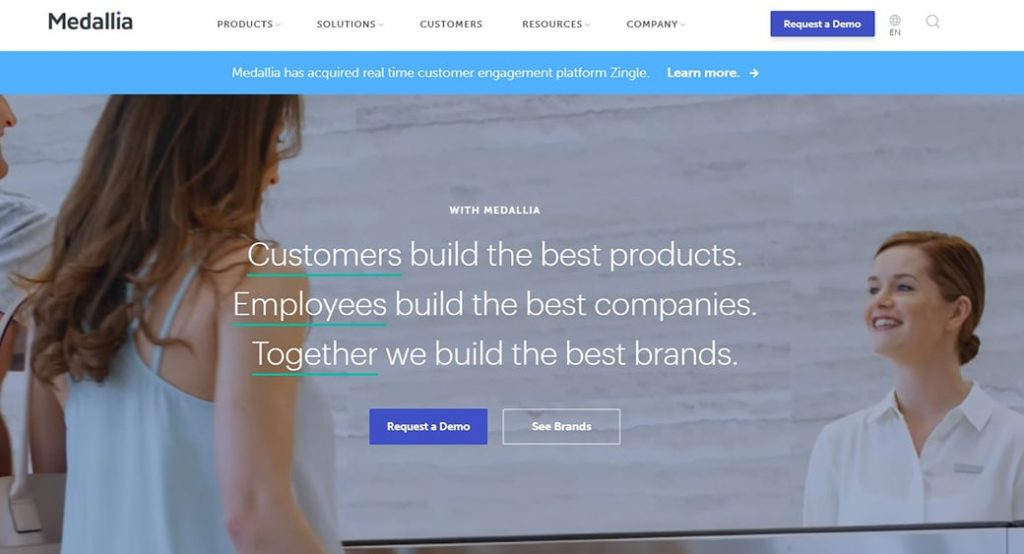This is a cropped screenshot of the Medallia website, showcasing the company's branding and recent acquisition. At the top left corner, the name "Medallia" is displayed prominently in large black font. Directly below, a vibrant blue banner spans across the width of the page, set against a background photo. Centrally placed within the banner, a text announces "Medallia has acquired real-time customer engagement platform Zingle," while to the right, a larger text invites visitors to "Learn More" with an accompanying right-pointing arrow.

The main background features a photograph of a woman smiling warmly from behind a desk, engaging with people standing in front of her. Superimposed on this background, in bold white font, the text reads: "With Medallia," followed by a motivational statement: "Customers build the best products. Employees build the best companies. Together we build the best brands." Notably, the words "customers," "employees," and "together" are underlined with an aqua-colored horizontal line for emphasis.

At the bottom left corner of the screenshot, a blue button labeled "Request a Demo" invites further interaction, while to its right, another option reads "See Brands". Additionally, a blue "Request a Demo" button is also visible at the top right of the page, ensuring visitors have multiple opportunities to engage with the site’s offerings.